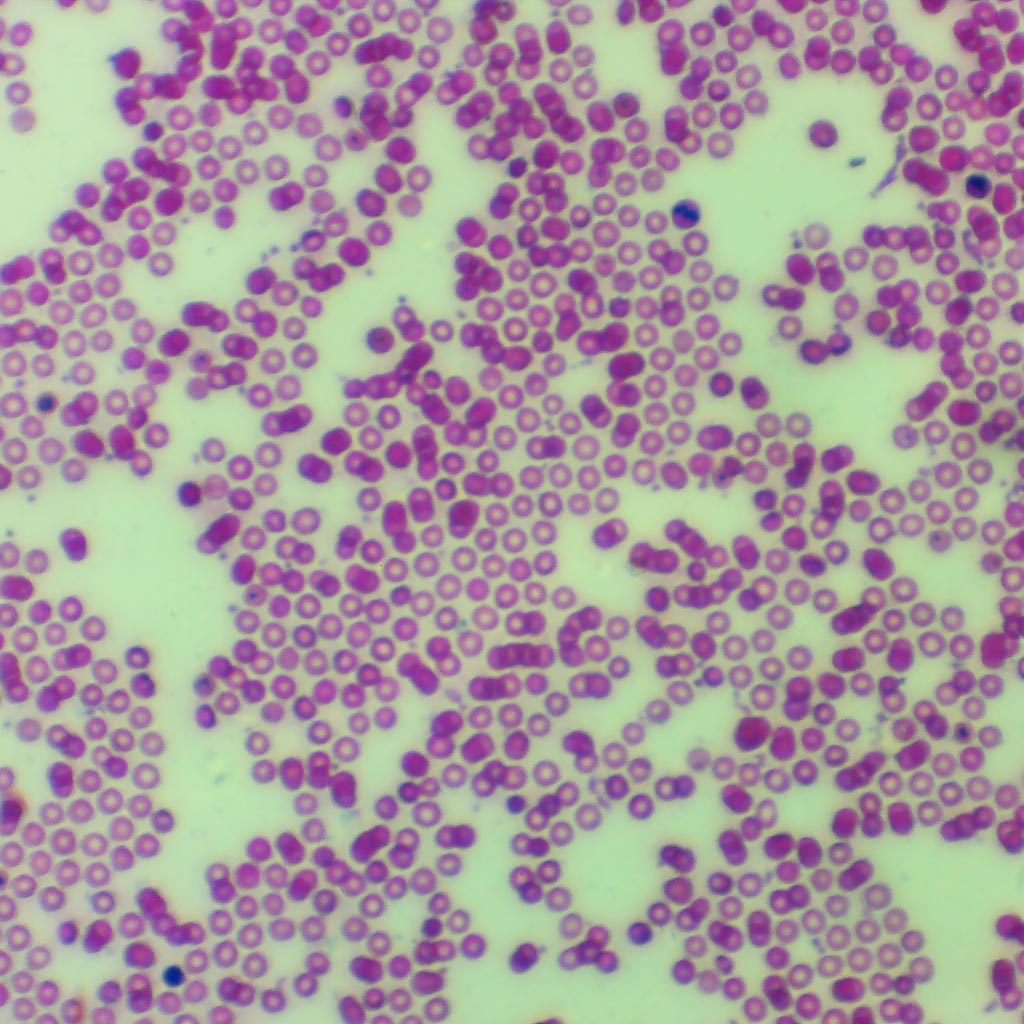The image appears to be a microscopic view showcasing numerous circular structures against a pea green background. These circles resemble amoebas or cells, varying in shades of purple—from light to dark—and some displaying blue dots. Scattered throughout the image, with no apparent pattern, these circles range in their opacity; some are hollow while others are filled. The depiction includes clusters of these circles, which number over a hundred, giving the impression of cellular or possibly blood-related elements. The intricate details of these purple and green structures make it suitable for scientific or biological contexts.